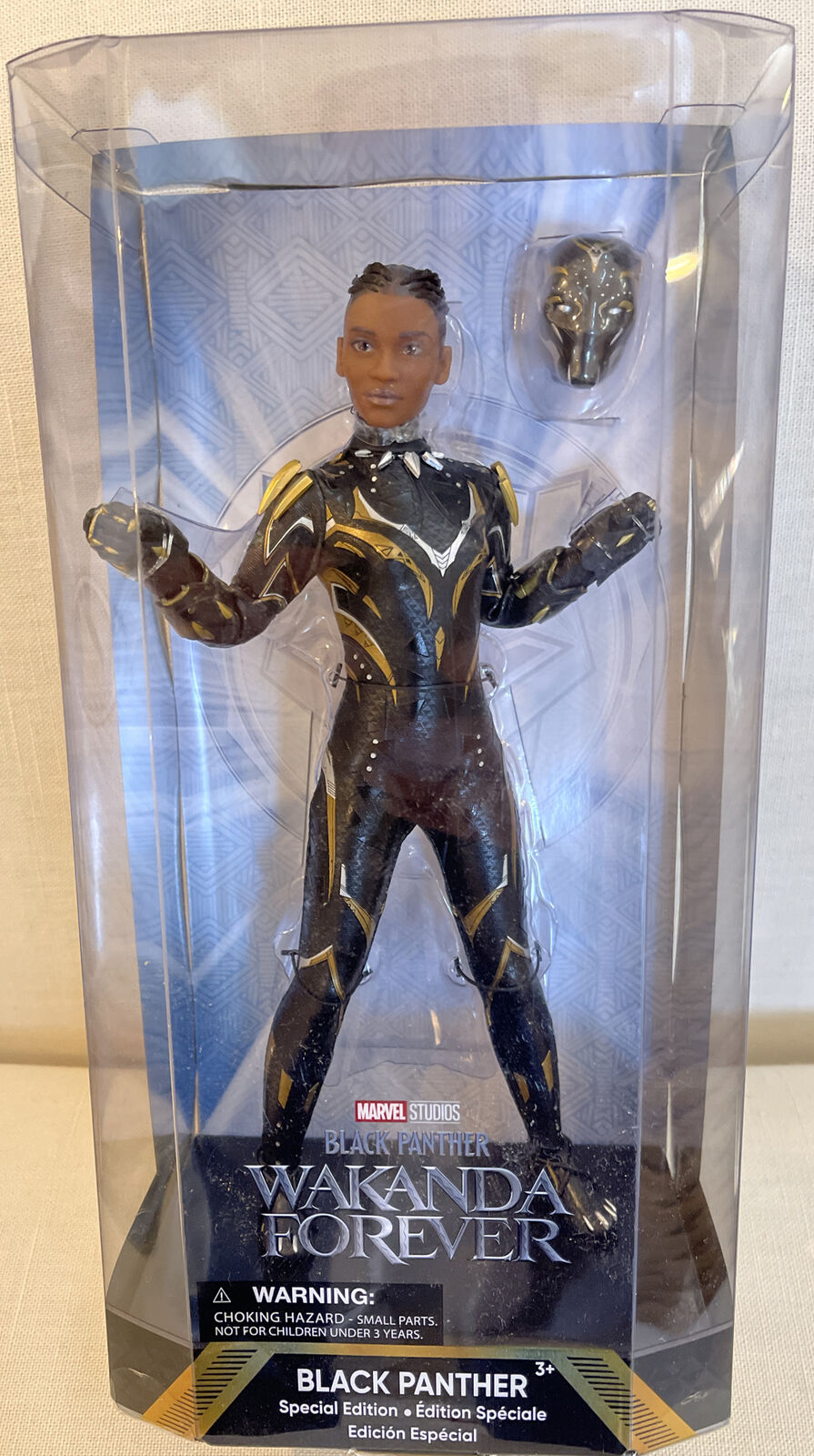This photograph captures a detailed look at a Black Panther action figure in its packaging, set against a beige wall and floor. The figure is encased in clear plastic packaging, backed by a sheet adorned with bluish-gray diamond designs. The action figure, a female character identified as the Black Panther, is dressed in a black skintight suit with gold stripes, and her hair is styled in cornrows, gazing off to the left. In the top right corner of the packaging, a Black Panther mask, featuring a black face, gold stripes, and silvery-white eyes, is mounted. The packaging prominently displays the Marvel Studios logo at the bottom front, followed by the text "Black Panther, Wakanda Forever." Below this, on a black box with white text, it warns: "Choking hazard, small parts, not for children under three years." At the very bottom, white text on a black background reads: "Black Panther 3 Plus Special Edition, Edición Especial, Edición Especial."